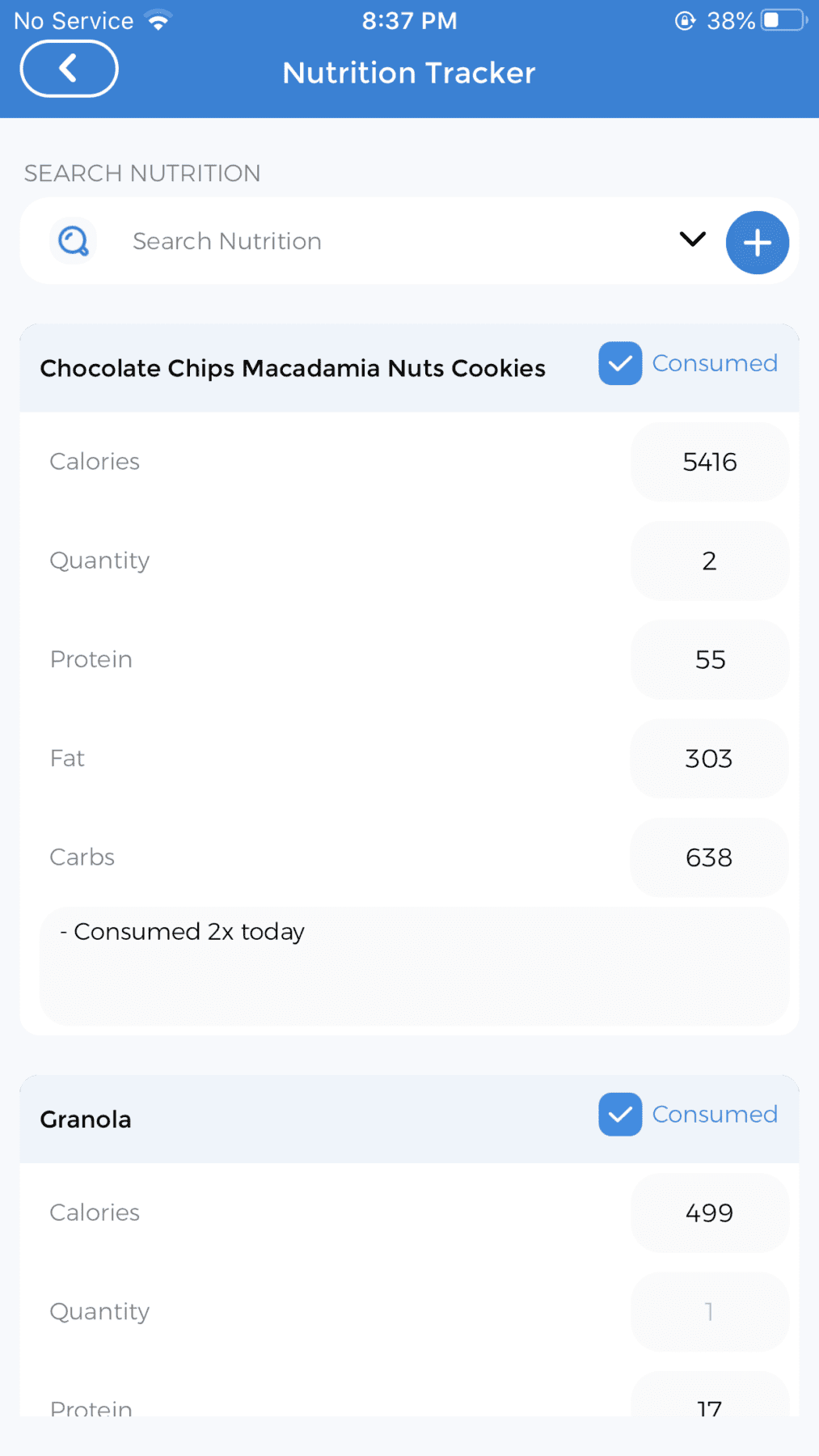The image is a screenshot of a nutrition tracker app displayed on a cell phone. At the very top, a blue banner spans horizontally. The top-left corner indicates "No Service" with an icon showing two bars of cell phone signal. The time reads 8:37 p.m., and the battery level is at 38%. Centered in the blue banner, the text reads "Nutrition Tracker."

Immediately below the banner, the page has a white background. A horizontal search bar spans across the page, with the placeholder text "Search Nutrition" displayed both above and within the search bar.

Underneath the search bar, bold text lists various food items. The first entry reads "Chocolate Chips, Macadamia Nuts, Cookies." Adjacent to this text on the right, there is a blue box with a white check mark, followed by the word "Consumed" in blue letters. Further details about this entry indicate the following nutritional information: 
- Calories: 5,416
- Quantity: 2
- Protein: 55 grams
- Fat: 303 grams
- Carbs: 638 grams
- Notation: "Consumed 2x today."

Below this, another entry, also in bold text, reads "Granola." Similarly, a blue square with a white check mark is to the right, followed by the word "Consumed" in blue text. The nutritional specifics provided for this entry are:
- Calories: 499
- Quantity: 1
- Protein: 17 grams.